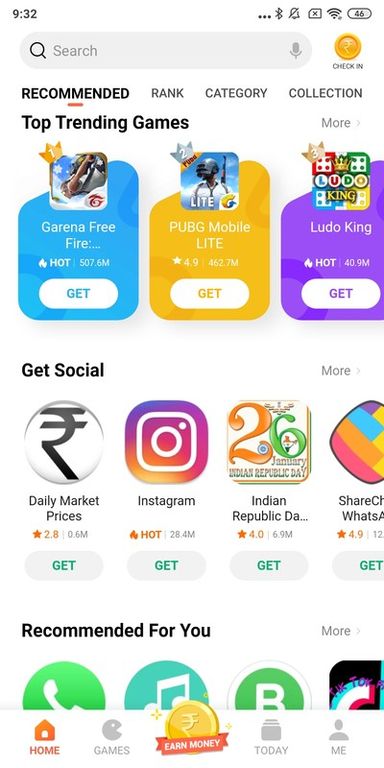The image depicts a mobile device screen with a white background. At the top of the screen, the time is displayed in black font as 9:32. To the right, there are three vertical dots indicating additional options for more information. Next to the dots, a black Bluetooth symbol indicates that Bluetooth is activated. Further right, an icon shows that notifications or sound are turned off, and the Wi-Fi signal is depicted as full. Additionally, the battery is shown to be at 46%.

Below the status icons is a gray search bar shaped like a rectangle with rounded edges, reminiscent of an oval with parallel sides. Inside the search bar, there is a black magnifying glass icon followed by the word "Search" in gray font, and a gray microphone icon.

Adjacent to the search bar is a yellow coin icon with the text "Check In." Below this area, in dark font, are labeled tabs: "Recommended," "Rank," "Category," and "Collection."

Further down, a black font heading reads "Top Trending Games," under which three games are presented. At the very bottom of the screen, the text "Get Social" is displayed.